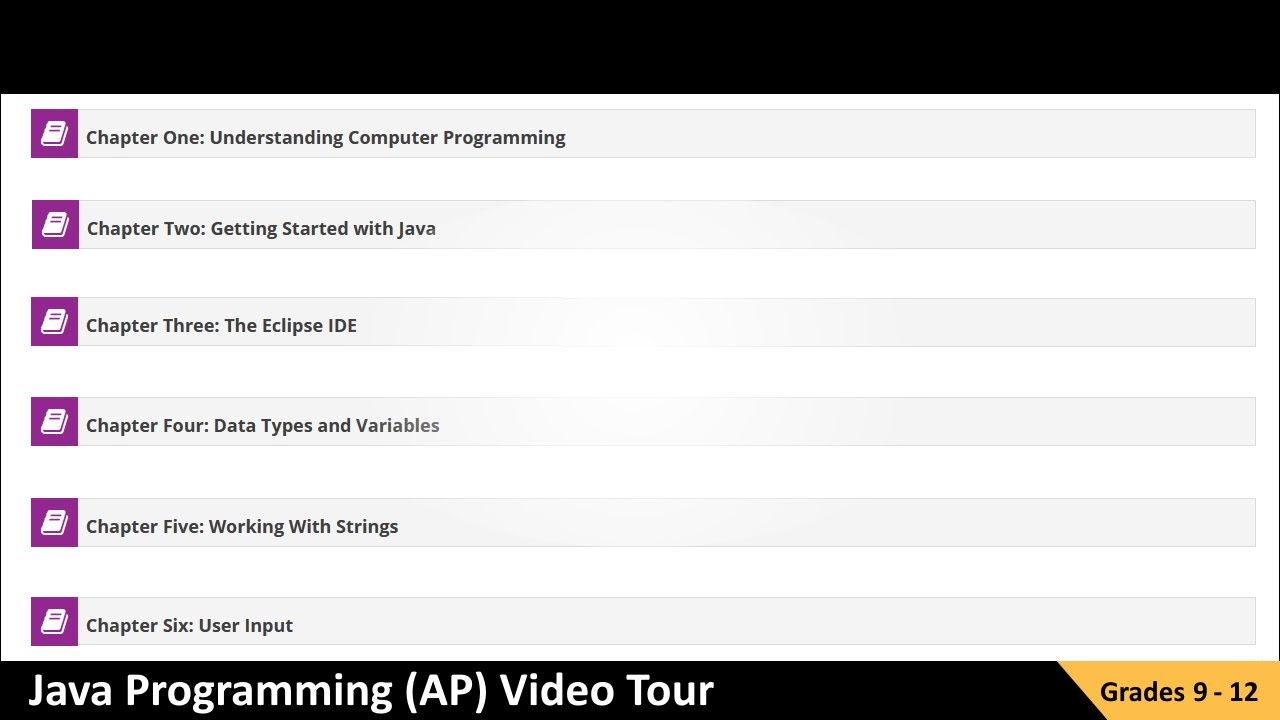The image showcases a structured layout for a Java Programming AP Video Tour, aimed at high school students in Grades 9 through 12. At the top and bottom of the image, there are black bars— the bottom black bar prominently features the title "Java Programming AP Video Tour," with a yellow-highlighted section stating "Grades 9 through 12" in the lower right corner.

The main content area is divided into six chapters, each detailing a key aspect of learning Java programming:

1. **Chapter 1: Understanding Computer Programming** 
   - Accompanied by a purple icon featuring a book, signifying it as the starting point.
   
2. **Chapter 2: Getting Started with Java**
   
3. **Chapter 3: The Eclipse IDE**
   
4. **Chapter 4: Data Types and Variables**
   
5. **Chapter 5: Working with Strings**
   
6. **Chapter 6: User Input**

The overall design is clean and minimalistic, dominated by white and black tones with occasional use of purple icons to visually demarcate different sections. This straightforward design underscores the educational focus of the material, guiding students through the fundamental concepts of Java programming.